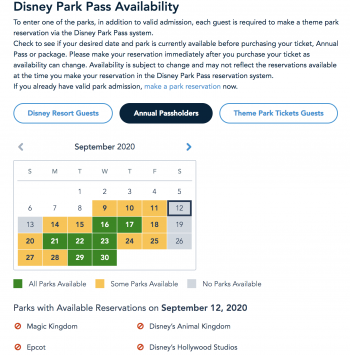A detailed screenshot of a Disney Park Pass Availability page. At the top of the page is the heading "Disney Park Pass Availability." Below this, a passage of text informs guests that to enter any of the parks, they must have both a valid admission and a theme park reservation made via the Disney Park Pass system. The text advises guests to check the availability of their desired date and park before purchasing tickets, annual passes, or packages, and urges them to make reservations immediately after their purchase since availability can change. 

Underneath this passage, there are three pill-shaped buttons labeled "Disney Resort Guests," "Annual Pass Holders," and "Theme Park Tickets Guests." The buttons for "Disney Resort Guests" and "Theme Park Tickets Guests" are white with blue text and outlines, while the "Annual Pass Holders" button in the middle is black with white text.

Below these buttons, a calendar grid displays various dates, marked in yellow, green, and gray squares, indicating different levels of availability for reservations.